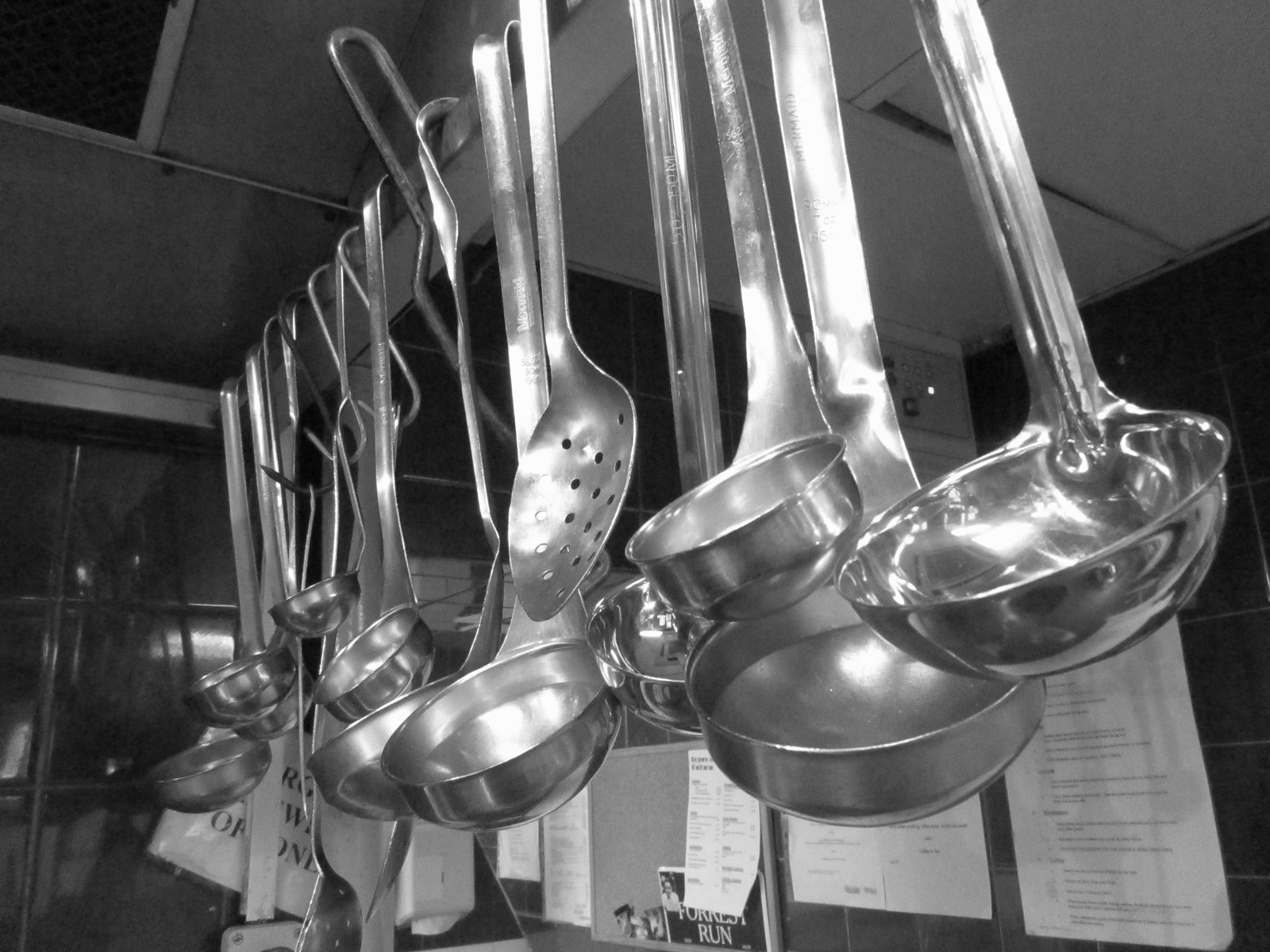A black and white photograph captures an intriguing view inside a kitchen, focusing on a collection of stainless steel ladles and cooking spoons. These utensils are suspended from a ceiling-mounted rack, with several of them hanging from S-hooks. Positioned at various lengths, there are approximately 10 to 15 ladles and spoons in total, featuring a mix of solid cups and one strainer spoon with perforations. The image is taken from a low angle, looking upwards, making the utensils appear large and prominent. The background reveals a dimly-lit room with papers and instructions posted on the walls. To the left, a window suggests nightfall outside. The overall setting hints at a professional kitchen or a restaurant’s back office, where these tools are essential for culinary tasks.